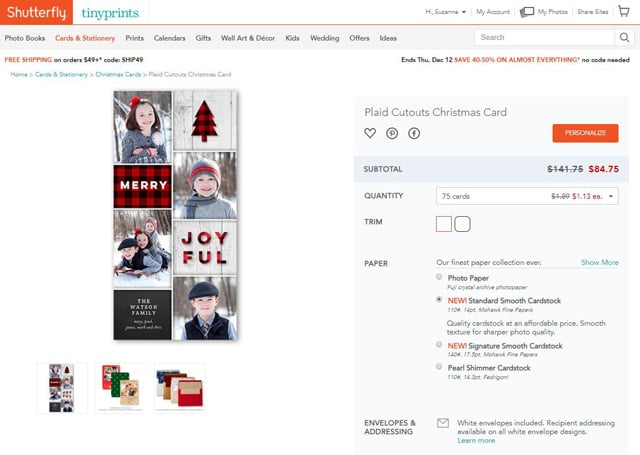The screenshot depicts a computer screen displaying Shutterfly's Tiny Prints section. Various product categories are visible, including Photo Books, Cards & Stationery, Prints, Calendars, Wall Art & Decor, Kids, Wedding, Offers, and more. A banner at the top announces free shipping on orders over $45 with the promo code SHIP49.

The user has navigated to the 'Cards & Stationery' section, where four card designs are displayed. One card features a photo of a little girl named Mary, while another shows a boy with a pine tree above his head. A third card depicts three children on a sled, and the fourth displays another child alone. Collectively, these cards represent the Watson family's Christmas card collection.

To the right of the screen, details about the selected card are shown: it's labeled "Plaid Cutouts Christmas Card." The order subtotal initially totals $141.75, but a 50% discount reduces the price to $84.75, which breaks down to $1.13 per card for a total of 75 cards. These cards are printed on the new Standard Smooth cardstock, and white envelopes are included. The site also mentions that recipient addressing is available for all white envelope designs. Overall, the Watson family's Christmas cards are ready for order completion.